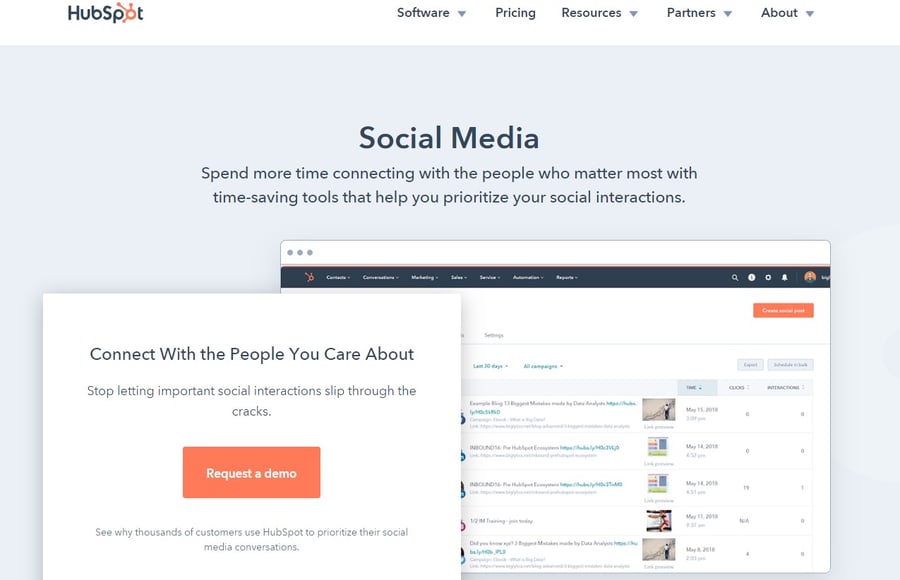Screenshot of a HubSpot Webpage: 

The image is captured from a desktop or laptop, evident from its wide dimensions. The screenshot is of a webpage without a visible URL bar. 

In the upper left corner, the HubSpot logo is prominently displayed, featuring the word "HubSpot" with the "O" rendered as an orange shape with tendrils. Adjacent to the logo, there is a white header with text links that include dropdown arrows for categories like "Software," "Pricing," "Resources," "Partners," and "About."

Below the header, the background takes on a light gray to light blue hue. Dominating the space are the words "Social Media" in large black text, followed by a tagline: "Spend more time connecting with the people who matter most with time-saving tools that help you prioritize your social interactions."

Beneath this text are two images. The first image displays the HubSpot interface. Overlaid on this is a prompt with a white background that reads, "Connect with the people you care about, stop letting important social interactions slip through the cracks." Below this prompt, there is a prominent orange button labeled "Request a Demo" in white text. 

This descriptive layout highlights HubSpot's focus on enhancing social media engagement through their platform's tools and features.